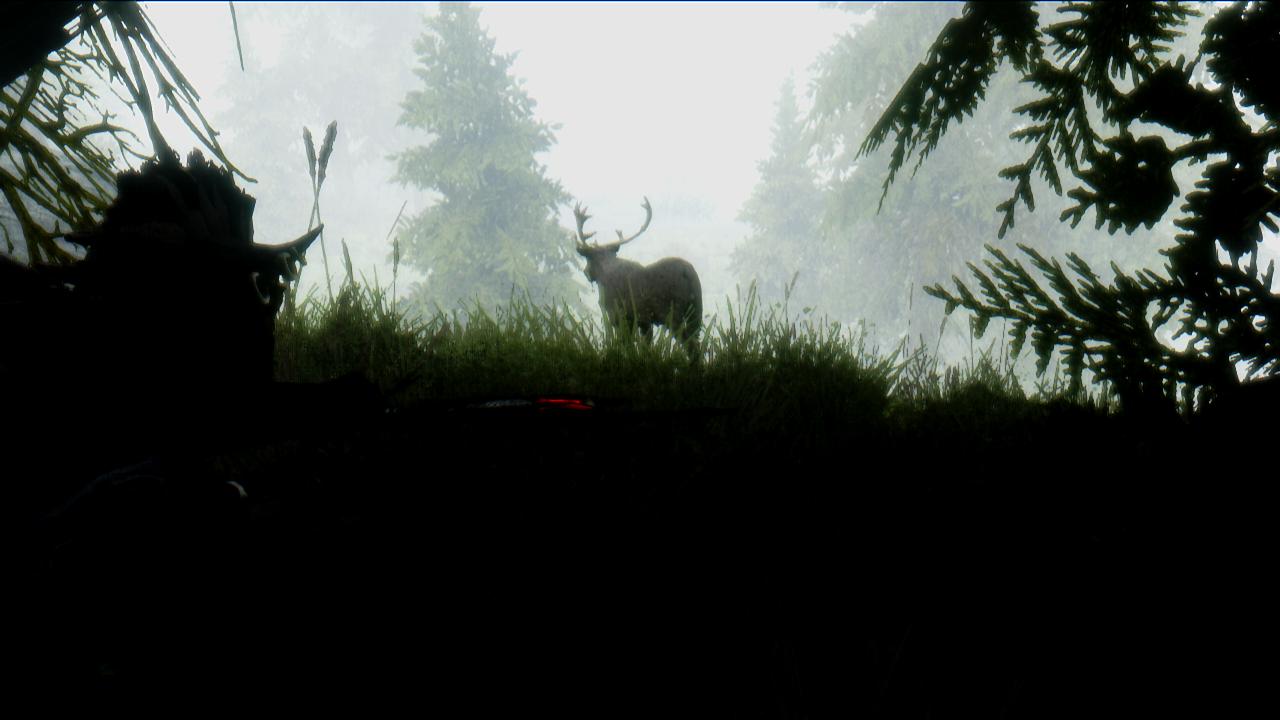In this captivating landscape photograph, we observe the back of a majestic moose framed by a foggy, light gray sky. The upper portion of the image reveals a serene, mist-laden atmosphere, contrasting with the dark green pine trees that fill the background, creating a sense of depth and isolation. The bottom half of the photo is shrouded in black, subtly grounding the scene. Patches of lush green grass peek through the natural framing provided by the silhouettes of trees on both the left and right edges, adding an element of intrigue and framing the majestic moose perfectly. The photograph, taken from behind the trees, exudes a mysterious and tranquil ambiance, capturing a moment of wilderness untouched by modern disturbances.